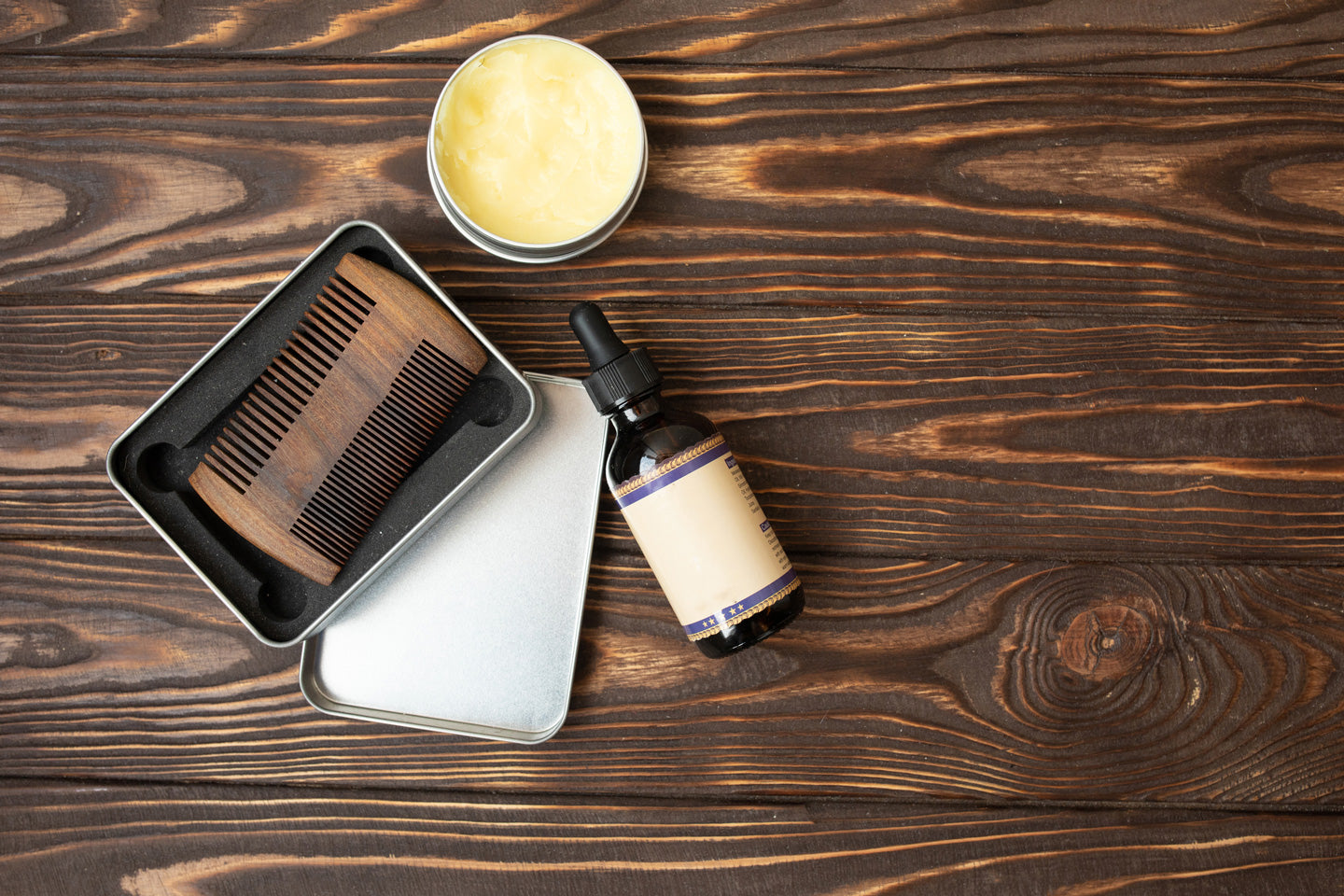The image features a meticulously staged setup against a rich, rustic wooden background, likely a table characterized by its raised, rough wood grain. Center-left dominates the focus, showcasing a round circular container filled with a yellowish ointment or goo. Adjacent to it, in the middle of the composition, there's an open rectangular tin case with a removed silver-colored lid placed underneath. Inside the tin case, nestled in black styrofoam, lies a unique wooden comb with teeth on both sides—the upper left teeth are wider spaced compared to the narrower teeth on the bottom right. Adding to the ensemble, an eyedropper bottle sits next to the tin, completing the array of items carefully arranged on the textured, dual-tone wooden surface.